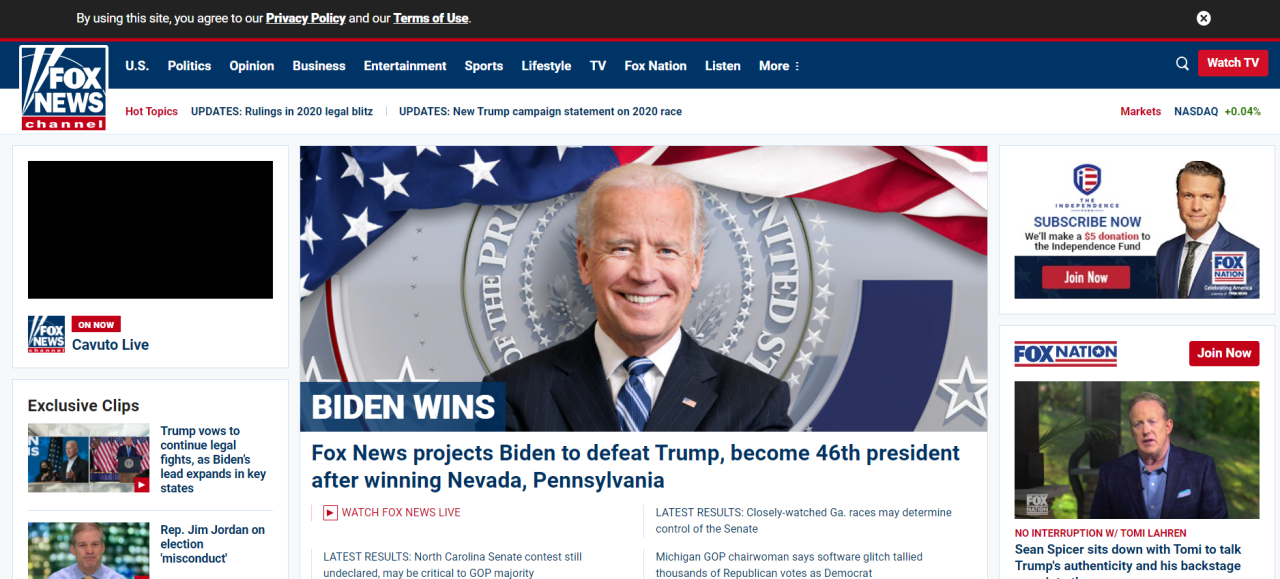The Fox News website on the night of the 2020 presidential election is prominently branded with its red, white, and blue logo labeled "Fox News Channel" in the upper left-hand corner. Adjacent to the logo is a dark blue navigation bar featuring white text for various links, including "US," "Politics," "Opinion," "Business," "Entertainment," "Sports," "Lifestyle," "TV," "Fox Nation," and "Listen." A "More" button with a dropdown menu appears at the far end of this toolbar. Housed on the far right of the navigation bar is a striking red button labeled "Watch TV," which redirects to the live TV feed.

Centrally positioned on the webpage is a prominent image of President Joe Biden. In the lower right corner of the image, a caption reads "Biden Wins." Below this, a subtext declares, "Fox News projects Biden to defeat Trump, become 46th president after winning Nevada and Pennsylvania," encapsulating the significant moment from the election night in 2020.